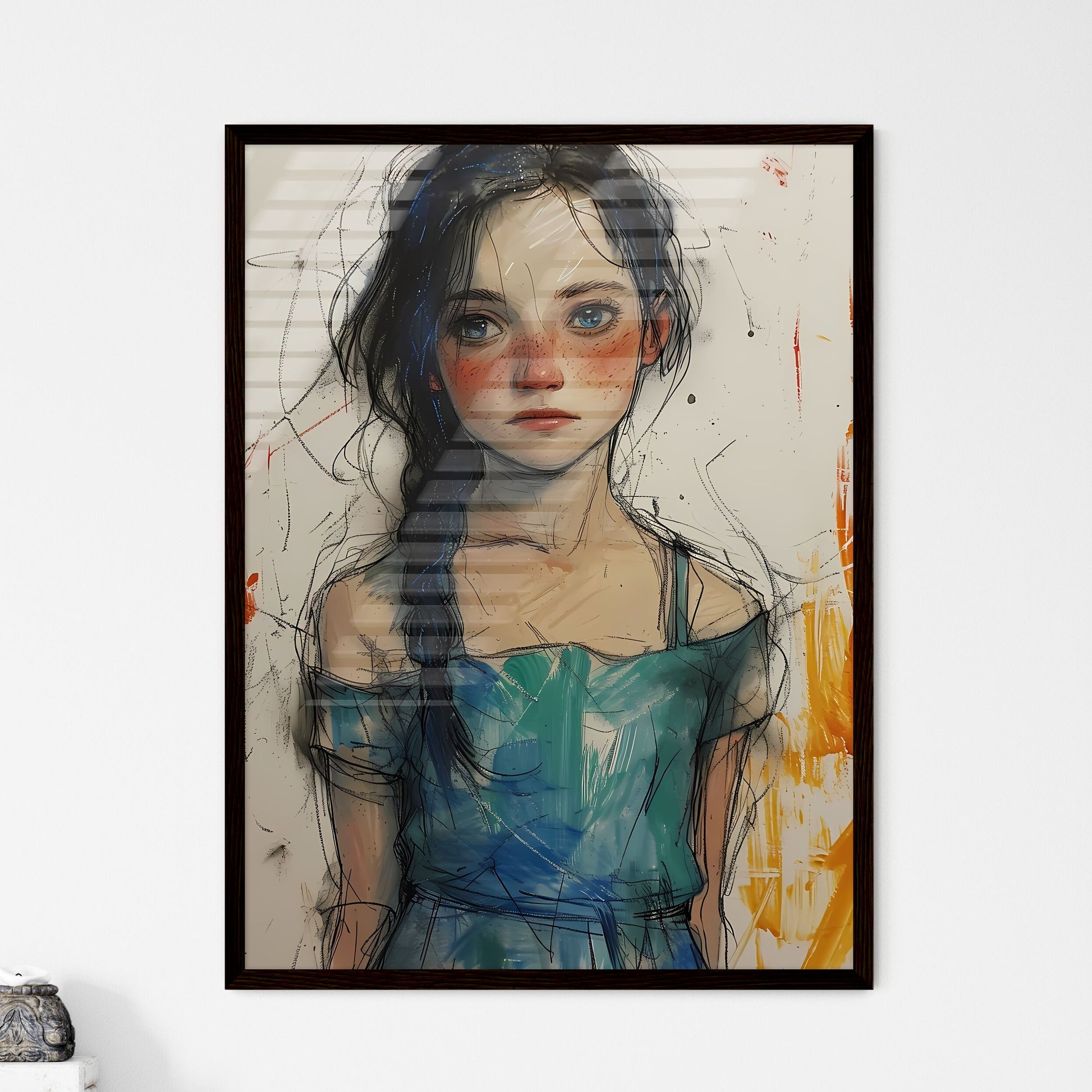In a gallery, a hand-drawn artwork of a teenage girl is framed with a thin, black rectangular border and mounted against a stark white wall. The girl, who has a cartoonish yet somewhat realistic look, has long, black hair tied into a scribbly ponytail that drapes over her right shoulder. Her blue eyes and rosy cheeks are accentuated by loose, unfinished brush strokes. She wears a blue and turquoise dress with one strap falling off her shoulder, adding to the sense of an incomplete piece. The background behind her features white slats that give the impression of a vertical window blind casting reflections. Small splashes of orange, yellow, and black paint scatter across the image, contributing to the painting's unfinished appearance. In the bottom corners, additional elements of the gallery setting are visible, including a small white platform that perhaps holds another object, enhancing the sense of the artwork's physical space.